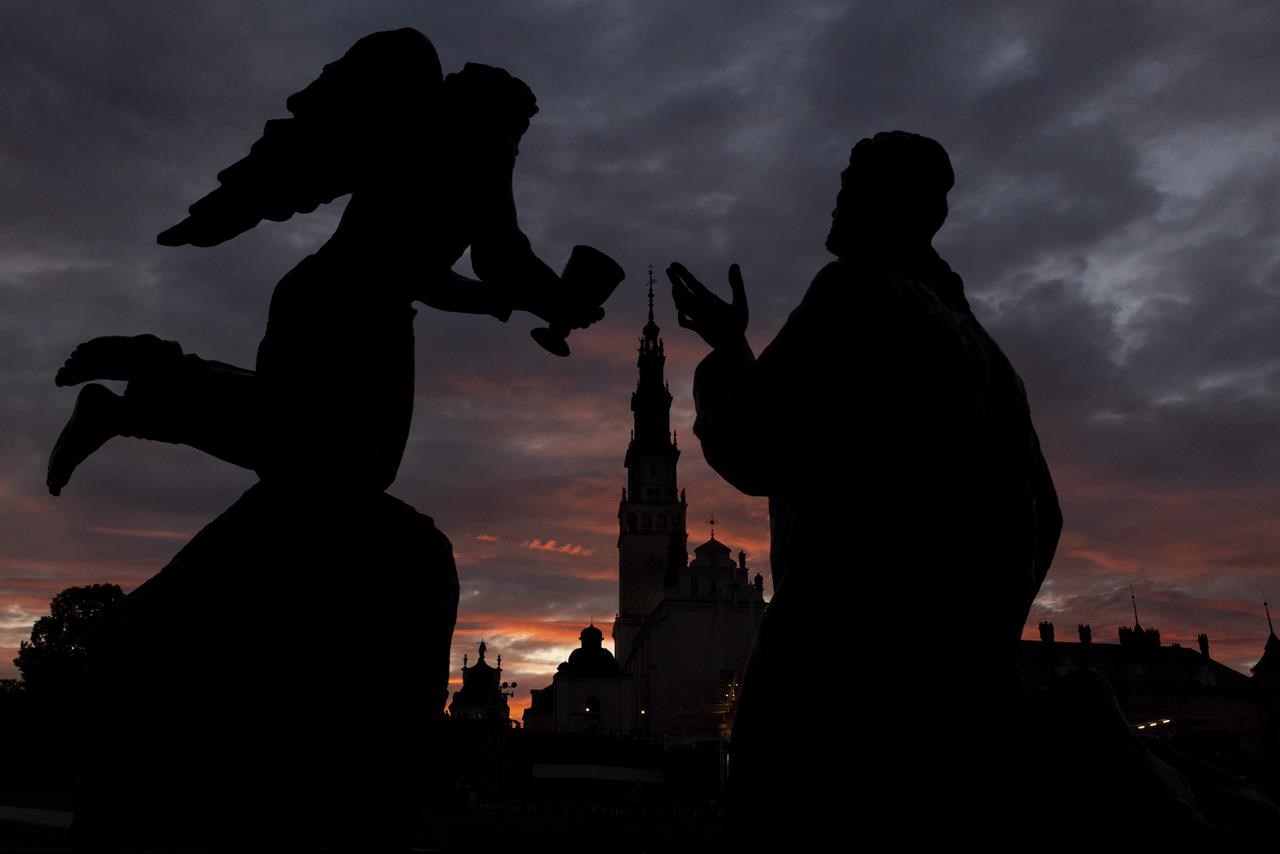The image depicts a dramatic evening scene somewhere in Europe, capturing the interplay of light and shadow at sunset. Dominating the foreground are two statues bathed in the twilight hues. To the right, a silhouetted figure resembling a man, stands with his hand raised, his features obscured in shadow. To the left, a kneeling statue of an angel with outstretched wings offers a cup toward the man. The angel appears perched on a rock, highlighting its serene posture. The background showcases an ornate cityscape with a large church featuring a tall steeple. The church's stained glass windows glimmer with a few scattered lights. Above, the sky is a canvas of striking pink, gray, and black clouds radiating outwards, enhancing the ominous yet beautiful ambiance. The scene is primarily rendered in a monochromatic palette with subtle hints of orange from the setting sun, adding a touch of warmth to the otherwise shadowy tableau.